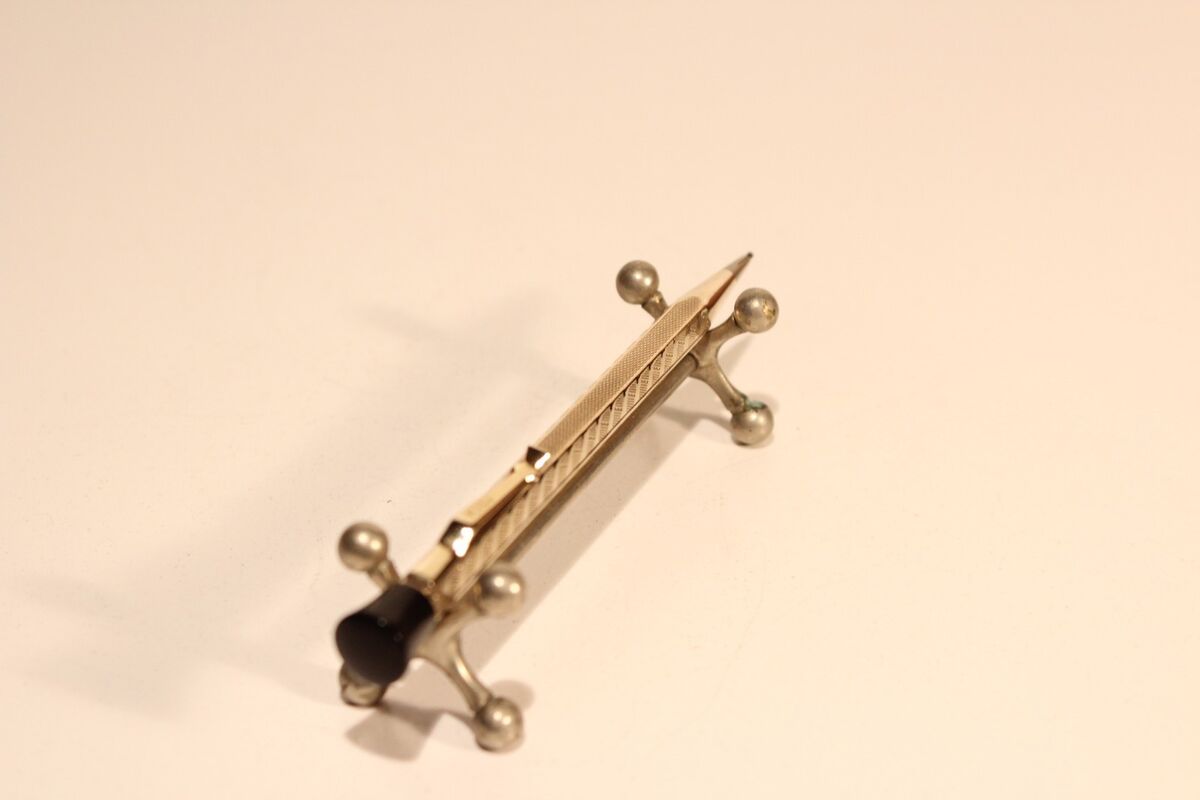The image features a metallic item set against an off-white or cream-colored background casting a slight shadow indicative of warm interior lighting. The primary structure consists of two brass-colored metal jacks, each with four small balls at the ends of the X-shaped arms, connected by a horizontal rod. Positioned atop this rod is a mechanical pencil with engraved texture for improved grip and a slightly extended lead at one end. The pencil is predominantly metal with a black end piece that includes a clip for attaching it to a shirt pocket. The overall appearance of the setup is reminiscent of a pen holder, designed with precision and detailed craftsmanship.